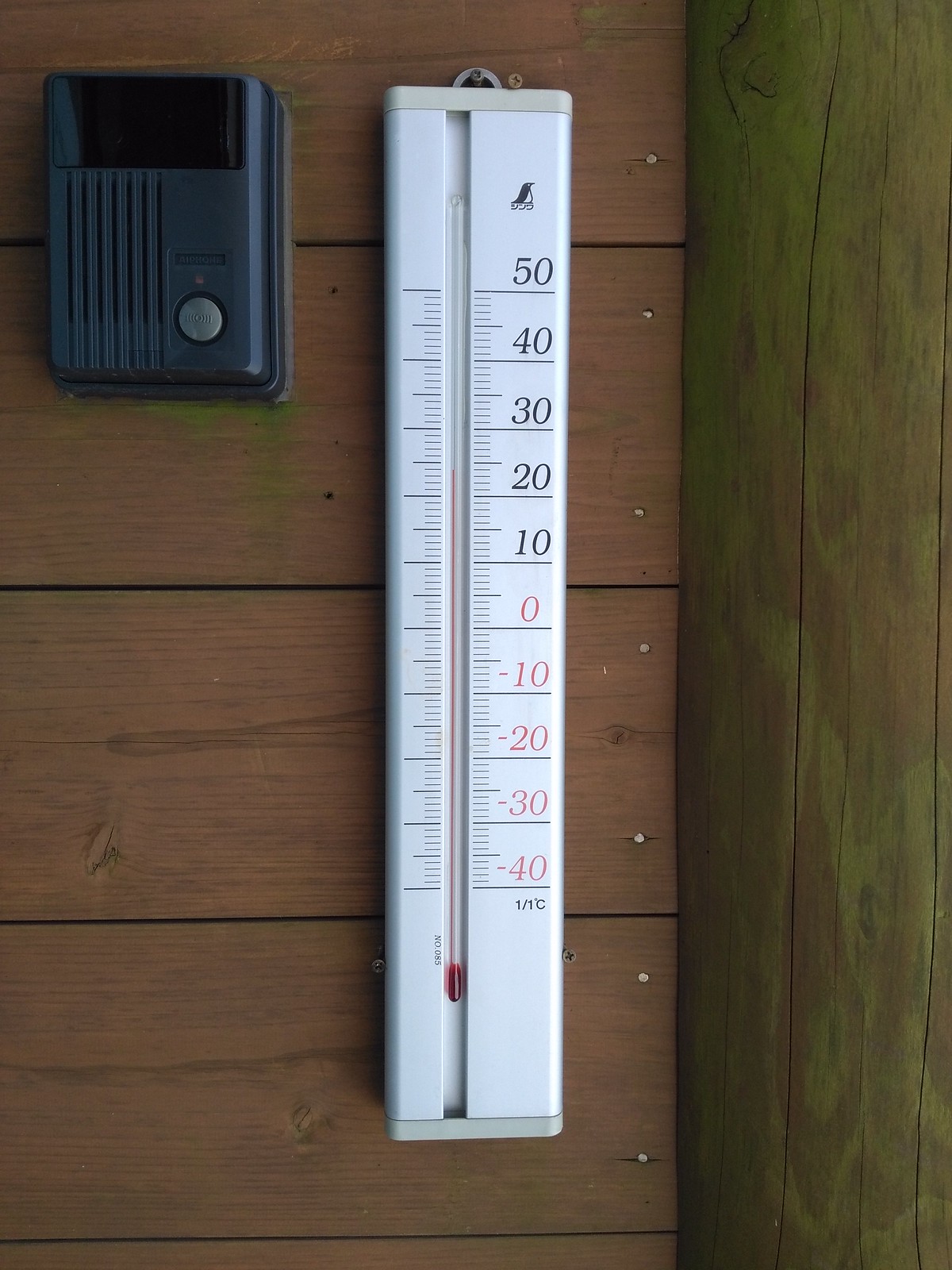This close-up image showcases a rustic wooden wall, revealing the fine details of the wood grain and visible nail marks on the weathered boards. Central to the composition is a white, plastic wall thermometer, suspended from a small hook. The thermometer, marked with temperature readings ranging from -40°C to 50°C, uniquely features red mercury, indicating the current temperature of approximately 24°C. Just below the thermometer is a rectangular, gray object, possibly a doorbell or an intercom speaker, adding to the practical yet worn aesthetic of the wall.